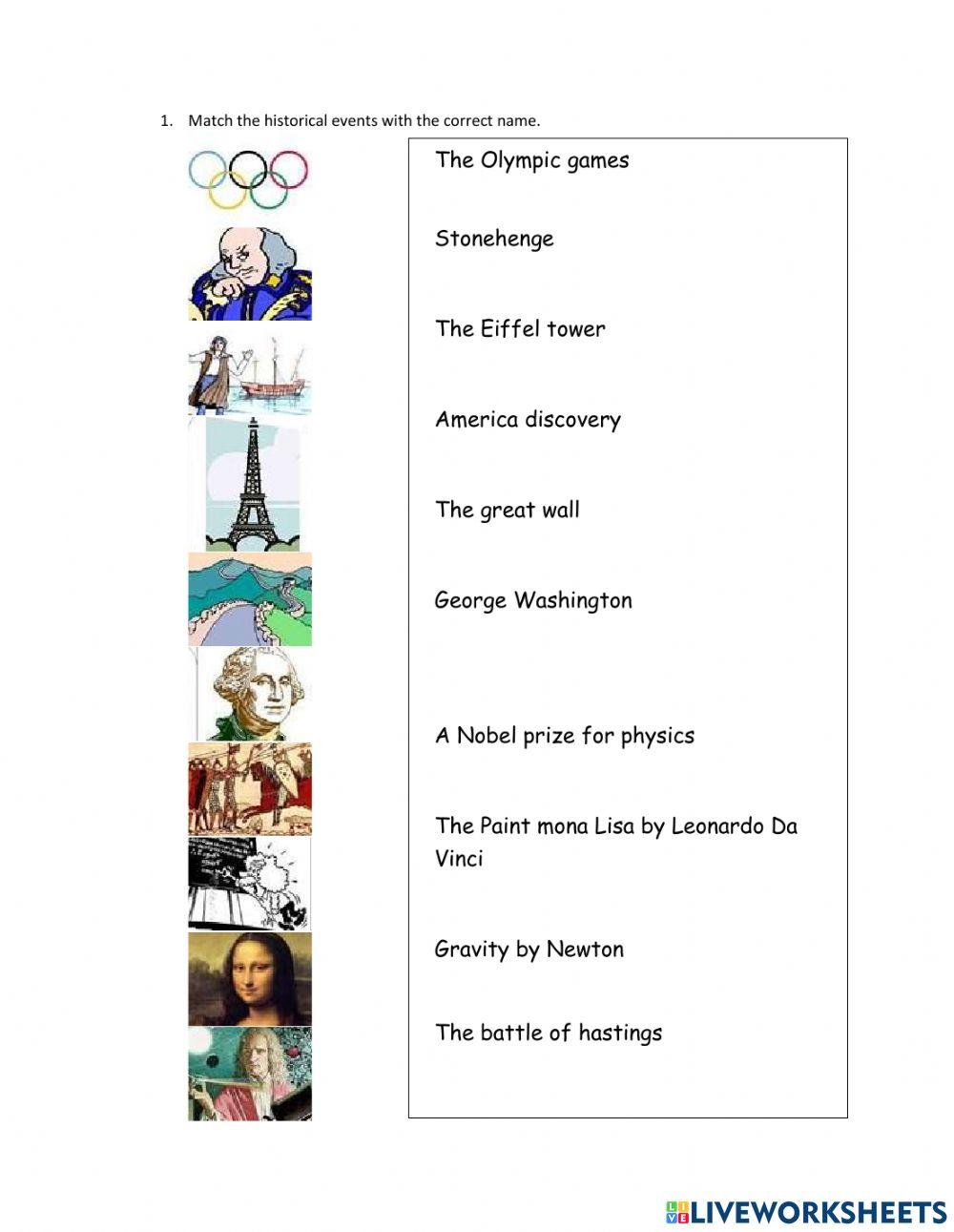This full-color vertical rectangular worksheet is designed to test your knowledge of various historical events and landmarks. At the top of the page, an instruction labeled "Number 1" states: "Match the historical events with the correct name." The left side features a series of cartoon-style images depicting famous scenes and figures, such as the Olympic rings, a king with gray hair, a boat in the harbor with a gesturing man, the Eiffel Tower, the Great Wall of China, George Washington, knights on horseback, a young student scribbling on a blackboard, the Mona Lisa, and Isaac Newton demonstrating his discovery of gravity. On the right side, there is a vertical column of names that correspond to these images, including the Olympic Games, Stonehenge, the Eiffel Tower, America Discovery, the Great Wall, George Washington, Nobel Prize in Physics, the Mona Lisa by Da Vinci, Gravity by Newton, and the Battle of Hastings. At the bottom right of the page is a blue logo that reads "Live Worksheets."